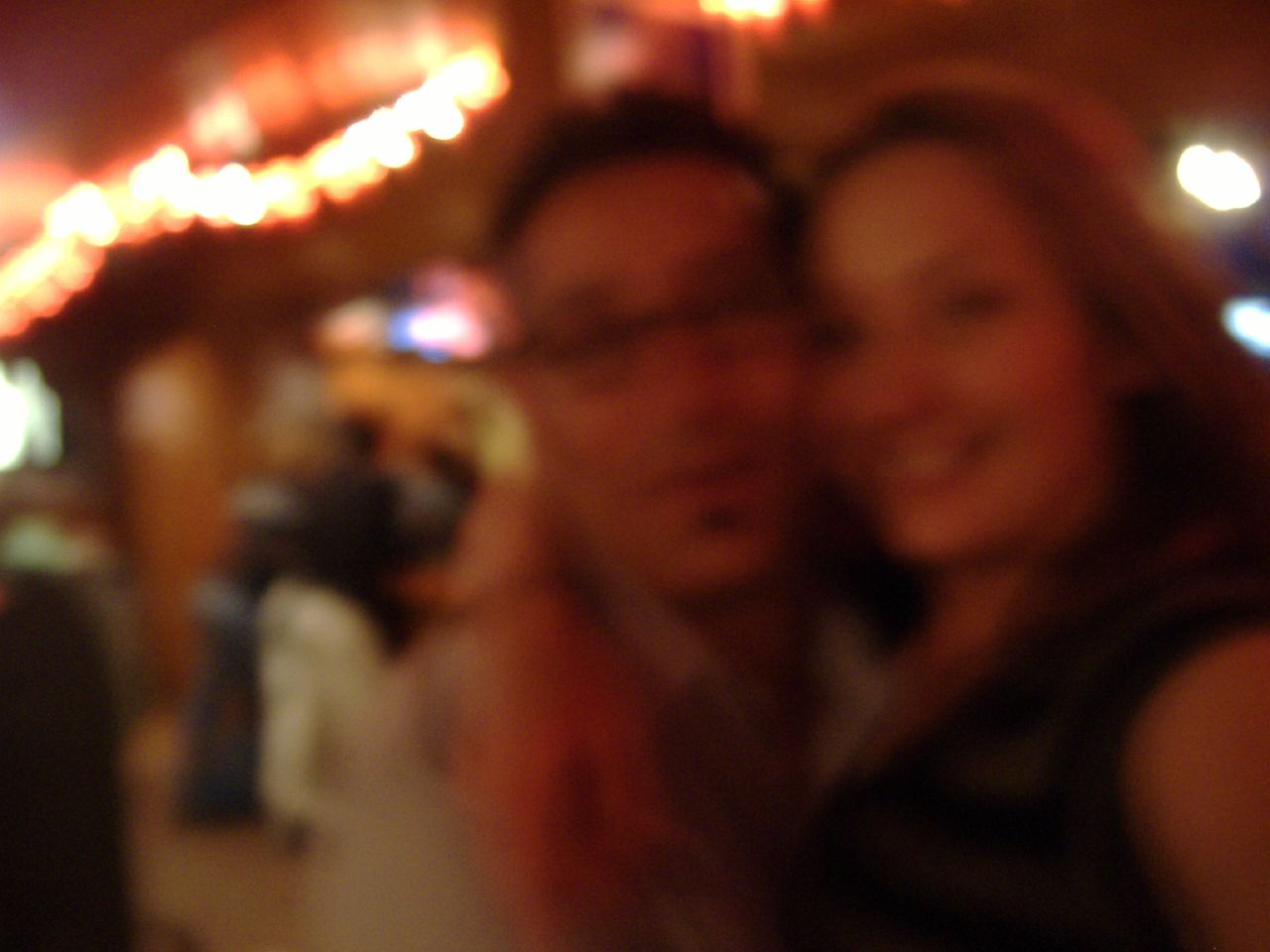In this slightly blurry photograph, a man and a woman are situated in the foreground, creating a focal point for the image. The man, who has dark hair, wears glasses and sports a small patch of facial hair on his chin. He is clad in a lighter-colored long-sleeve shirt. The woman beside him has long brown hair and is captured smiling brightly. She is dressed in a short-sleeve black and gray striped shirt and has her arm affectionately draped around the man's neck. 

The background of the photograph features a cozy setting adorned with festive decorations; white Christmas lights hang intricately on a wooden wall. The walls have a wood-toned finish while the floor is tan-colored, contributing to the warm ambiance. Additional figures populate the background, including a person in a dark shirt and white pants, and another individual in a darker shirt paired with jeans. Also visible are several blurred lights and what appears to be a television, adding layers of depth to the scene.